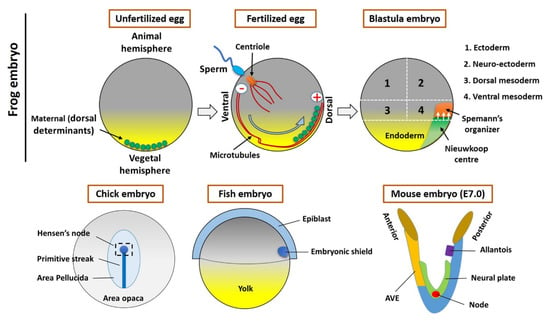This detailed diagram illustrates the developmental stages of a frog embryo, transitioning from an unfertilized egg to a fertilized egg, and eventually to a blastula. It begins with an unfertilized egg labeled "frog embryo," showing "maternal dorsal determinants" marked by green circles in the vegetal hemisphere and the "animal hemisphere" facing upward. The "fertilized egg" stage is depicted with a sperm outside the egg and a centriole, resembling an octopus-like structure, inside. Microtubules extend between the ventral and dorsal regions, guiding the developmental process.

The blastula stage is broken down into four distinct components: "1. Ectoderm," "2. Neuroectoderm," "3. Dorsal Mesoderm," and "4. Ventral Mesoderm," illustrating the differentiation of cell layers. Additionally, essential aspects like "Spemann's organizer" and the "Nieuwkoop center" are highlighted.

Beyond the frog embryo, the diagram encompasses comparative developmental stages of other species: "chick embryo" with "Henson's node," "primitive streak," "area pellucida," and "area opaca"; "fish embryo" at the "blastula" stage with an "embryonic shield"; and "mouse embryo" at stage "E7.0," detailing "anterior," "posterior," "allantois," "neural plate," and "notochord."

Each embryo's depiction—using gray circles and yellow coloring for the yolk—provides a visual comparison of embryonic development across different species. This comprehensive diagram serves as an educational tool to understand the intricate processes and stages in embryogenesis.